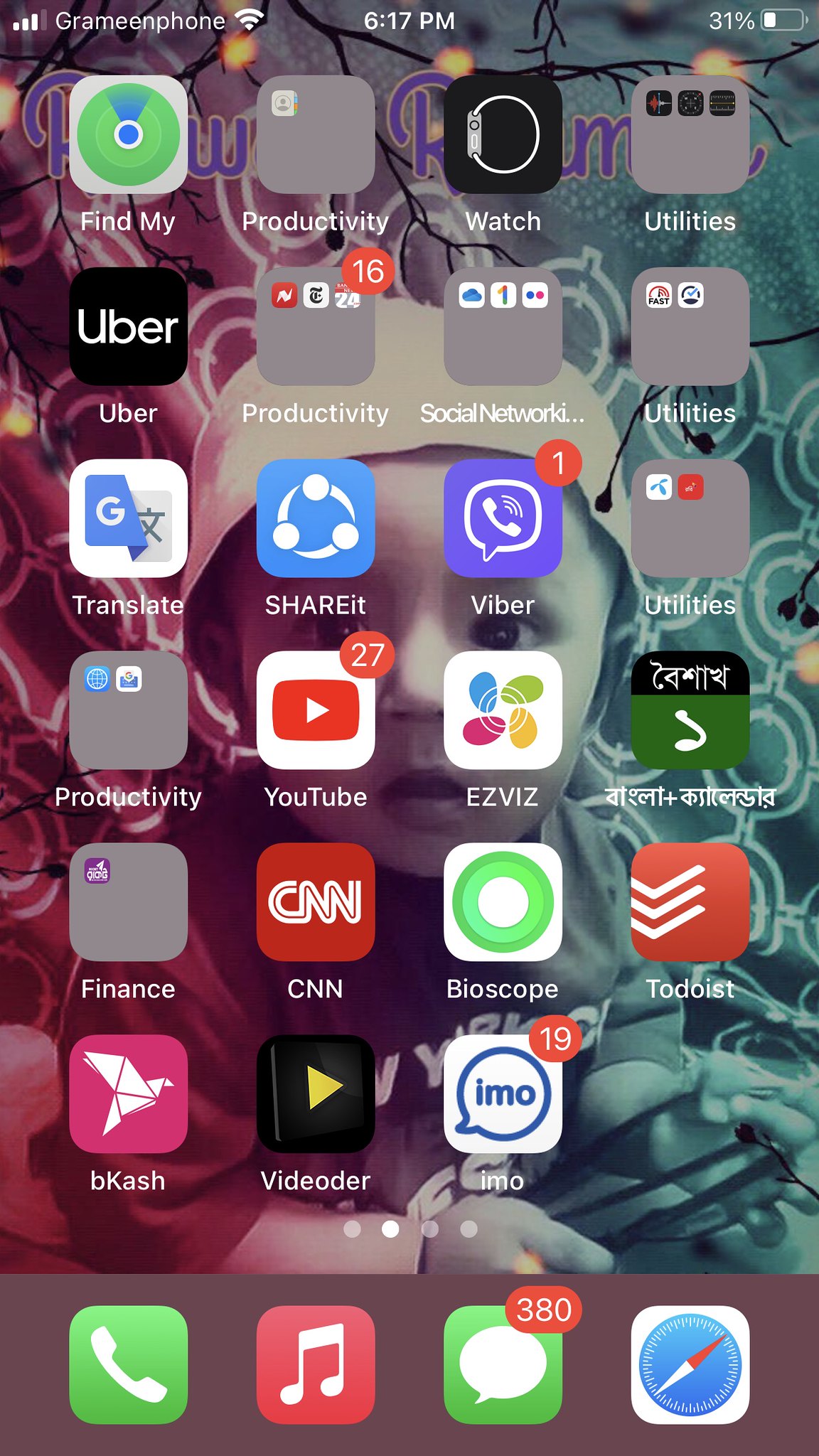The home screen of this iPhone features an endearing wallpaper of a baby, likely a relative of the phone's owner. The interface is organized into several folders and individual apps. Prominently, there are folders such as Productivity, Social Network, three Utilities folders, and multiple additional Productivity folders, demonstrating a structured approach to app management. A Finance folder is also present. 

Among the standalone apps, notable ones include CNN, Uber, Apple Watch, and Google Translate. The dock at the bottom houses essential apps: Phone, Music, Messages, and Safari.

The notification center is bustling with activity: Messages has 380 unread texts, YouTube shows 27 notifications, Viber has one, and a Productivity folder contains 16 alerts. The time displayed is 6:17 PM, the battery is at 31%, and the device is connected to Wi-Fi with the network named "gramophone." It's a typical yet visually organized iPhone home screen, offering a glimpse into the user’s digital life.